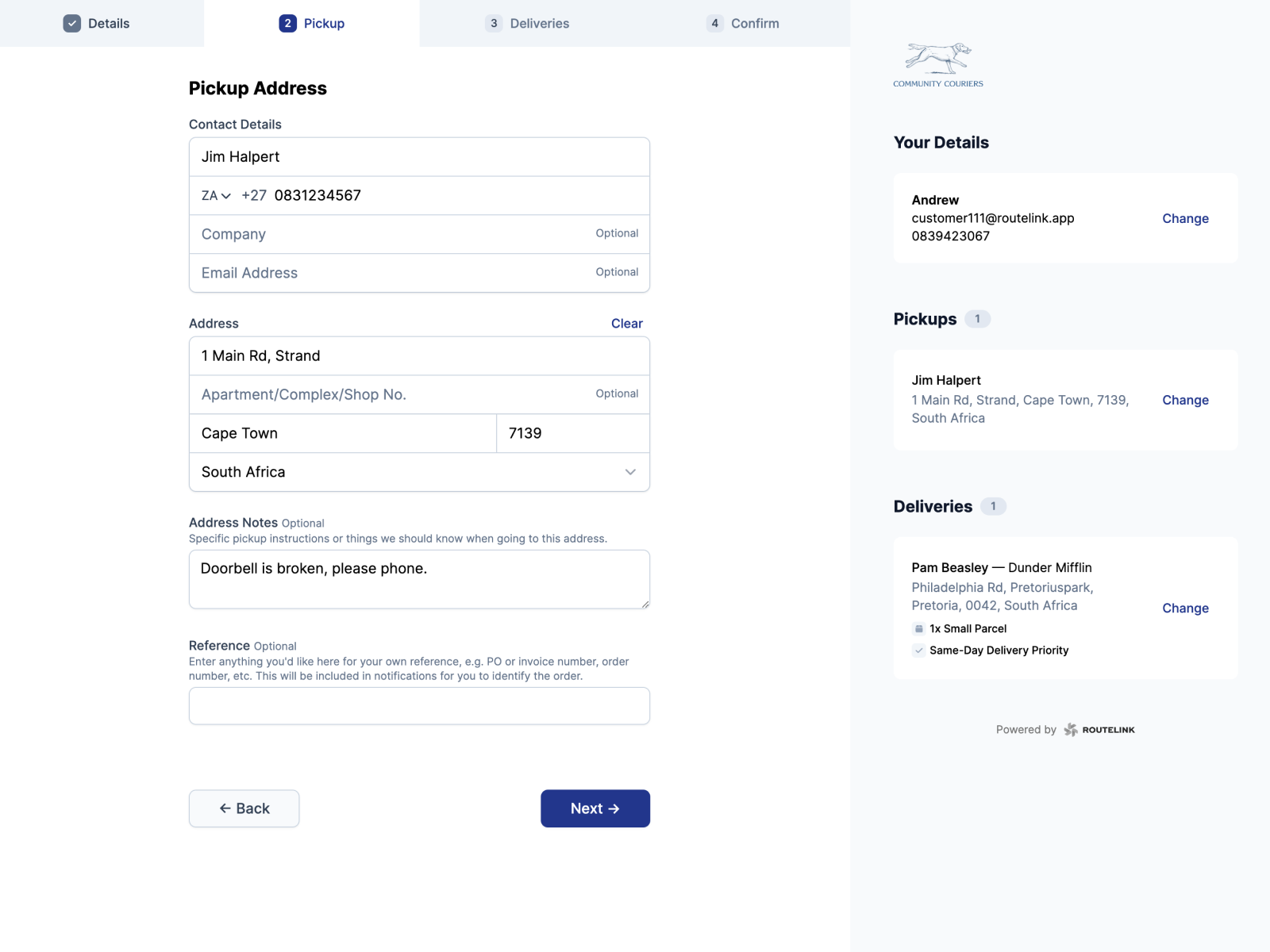A detailed example on a South African courier service website illustrates how to place an online delivery request. The sample page uses characters from the TV show "The Office" for clarity. Here, Jim Halpert is arranging a pickup for a package from his listed address, located on Main Road in Strand, Cape Town, South Africa. Despite Jim Halpert being a fictional character from Scranton, Pennsylvania, this example helps users understand the process. The package is intended for delivery to Pam Beasley, Halpert's fictional girlfriend, at Dunder Mifflin Paper Company. The scenario even includes specific instructions for the courier: Jim Halpert's doorbell is broken, so the delivery person should phone him upon arrival. This illustrative approach offers a clear and engaging way for users to learn about the courier service's functionalities.